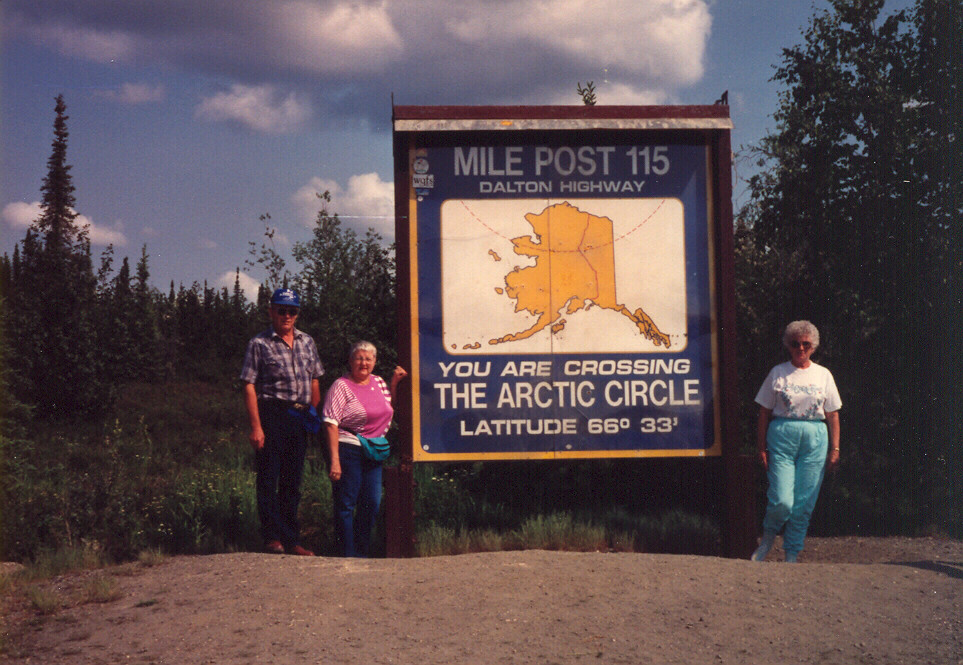The photograph, likely taken in the seventies or eighties, depicts three elderly people—a man and two women—posing in front of a large sign that reads "Mile Post 115, Dalton Highway, You Are Crossing the Arctic Circle, Latitude 66°33'." The atmosphere suggests it is summertime, with all three individuals dressed in short-sleeved shirts: the man in a button-down plaid flannel shirt tucked into blue jeans paired with brown boots, one woman in a pink shirt and blue jeans, and the other in a white shirt and light blue joggers. They are standing in a scenic, forested area, possibly a national park, enjoying their vacation. The day appears mildly cloudy but overall pleasant, underscoring the warmth and tranquility of the moment. The impressively tall sign stands prominently behind them, marking the significant geographical location.